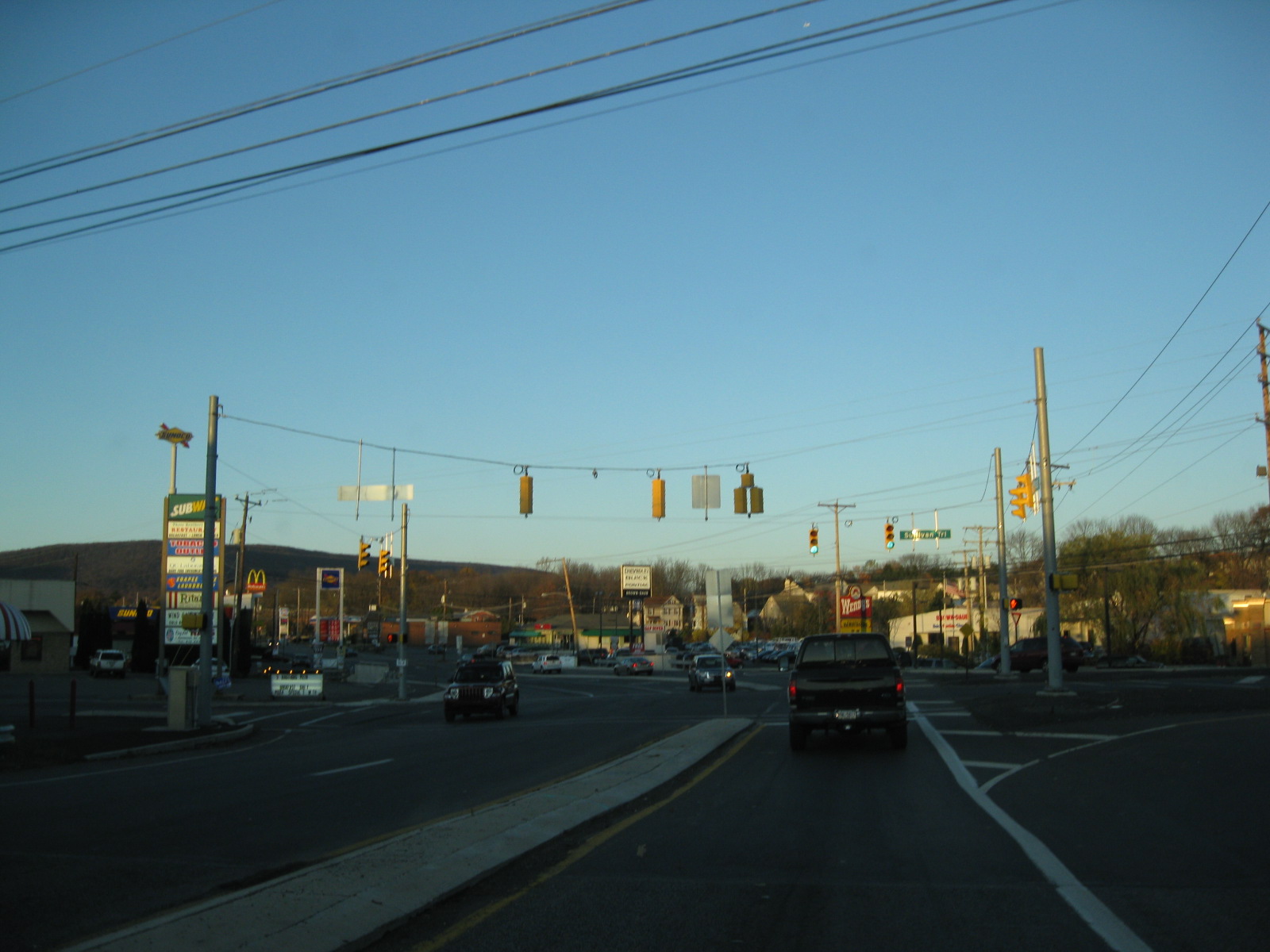This photograph, taken from the interior of a car, captures a bustling urban street scene at what appears to be a four-way stop. The car is positioned directly behind a pickup truck, waiting at a traffic intersection. Overhead, traffic lights hang and currently display a green signal. On either side of the street, a series of shopping strip malls dominate the scene, with a variety of eateries visible. To the right, the iconic Wendy's sign suggests an approaching fast-food restaurant. On the left, the recognizable yellow arches of McDonald's and a Subway sign indicate additional dining options. The photograph shows a mix of vehicles traveling in both directions along the road—three are particularly notable: two approaching the camera and one heading away from it. The image embodies a typical snapshot of city life, characterized by commercial activity and steady traffic flow.